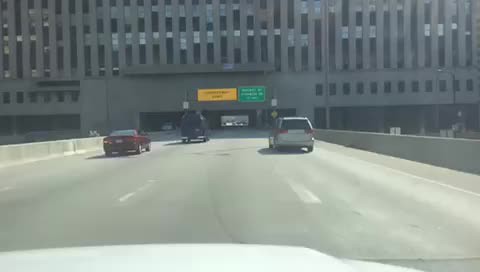This color photograph, taken from the perspective of the driver inside a white vehicle, showcases a bustling four-lane highway heading towards a large concrete tunnel beneath a Brutalist-style building. The image captures the view through the windshield, with the white car positioned in the second lane from the right. The highway appears to be designed with at least four lanes in each direction, making it an eight-lane thoroughfare in total. The scene is well-lit with bright daylight illuminating the highway from the upper right, casting slight shadows.

In the foreground, the white hood of the vehicle is visible, adding to the sense of immersion. To the left of the white car, a variety of other vehicles populate the highway: a silver SUV, a green van, and a red sedan are heading towards the imposing concrete structure. This multi-story building features vertical gray columns with windows nestled between them, creating a distinctive architectural appearance. As the road approaches the tunnel, concrete barriers line the sides, with both yellow and white dotted lines demarcating the lanes.

The distant tunnel entrance and exit are visible, framed by street signs suspended above them. Although the text on these signs is not legible, their positions are noted: a long yellow rectangle sign to the left and a green rectangular street sign to the right. This detailed imagery captures both the dynamic nature of the highway and the architectural elements of the surrounding infrastructure, providing a comprehensive view of the scene.